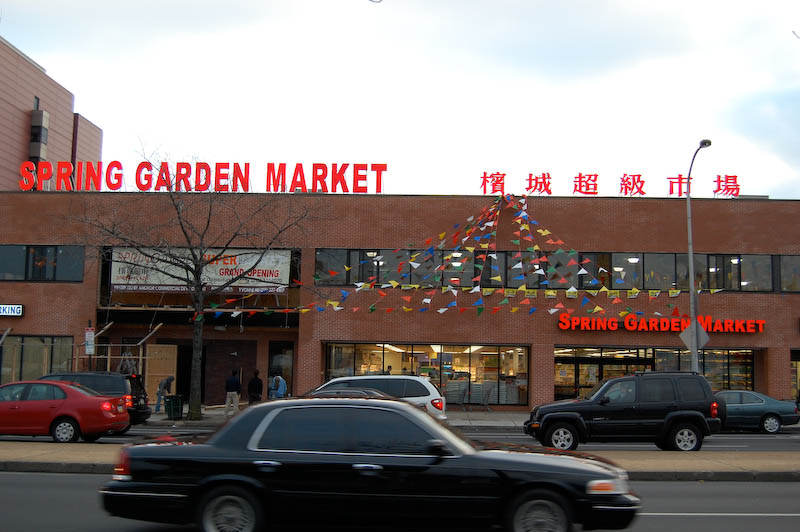A photograph captures a bustling urban street scene featuring the two-story red brick building of Spring Garden Market. Prominently displayed at the top of the building, the market's name is illuminated in large red letters, accompanied by inscriptions in an Asian language, possibly Chinese, to the right. Below, colorful pennant flags in shades of red, yellow, blue, and green drape from the roof, suggesting a cheerful event, perhaps a grand opening. The street in front of the market is lively, with multiple cars, including a black car, a red car, a silver or white van, a green car, and another black car, some parked and others driving by. People are seen walking near the entrance on the left side of the image, adding to the dynamic atmosphere. A street lamp stands at the bottom right, further framing the scene of this vibrant market storefront on a clear day with a light blue sky, hinting at either dawn or dusk.